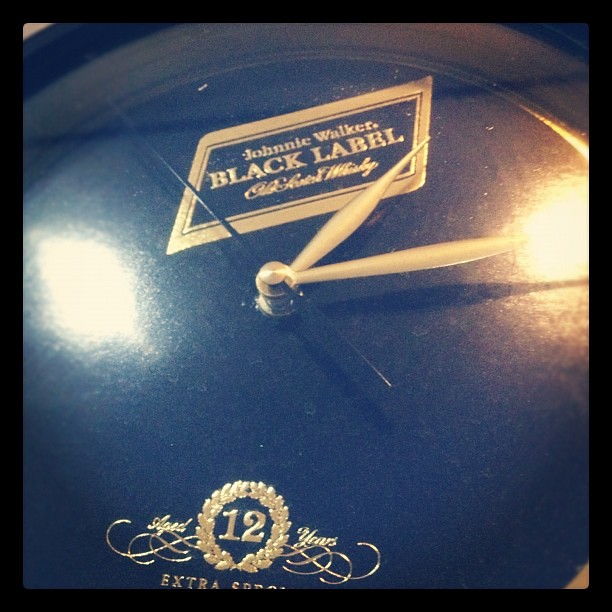This detailed close-up captures a luxurious, reflective black clock face that serves as an advertisement for Johnny Walker Black Label whiskey. The clock itself is striking in its simplicity, devoid of any numerical markings. Instead, the smooth, glossy black surface is accentuated by the reflection of two bright light spots, which add a dramatic flair. The clock's hands are elegantly crafted in gold, contrasting sharply with the sleek, black second hand. The time displayed is approximately 2:15. Dominating the lower portion of the clock face, just above the position where the six would normally reside, is the iconic Johnny Walker Black Label branding. This is rendered in opulent gold with meticulous lettering, proclaiming "AGED 12 YEARS" in an ornate gold leaf design flanked by laurel embellishments. Beneath this, the word "EXTRA" is prominently featured in bold, gold letters, further emphasizing the premium quality of the whiskey.